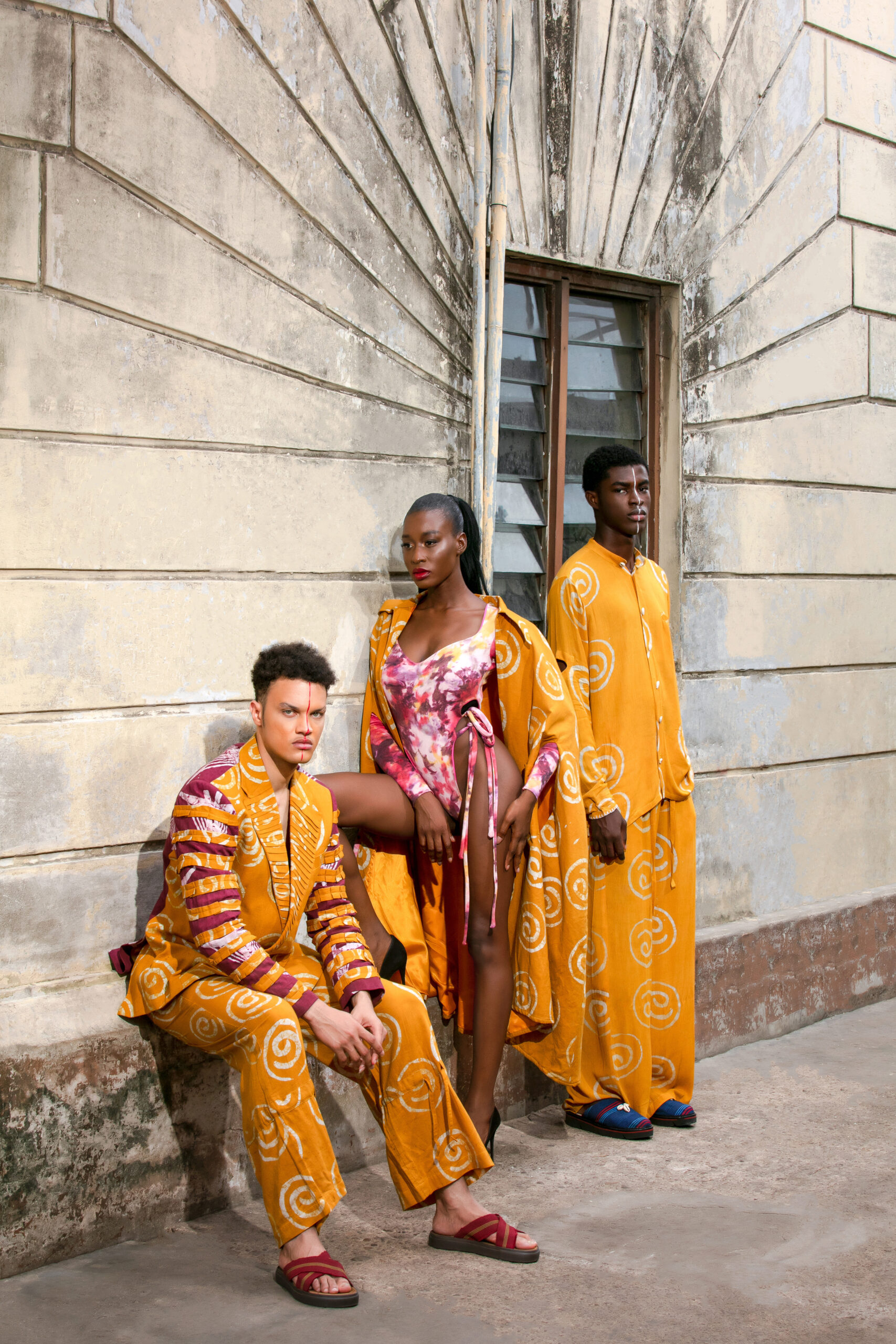In this photograph, three individuals are seen outside a white building characterized by a rectangular window with multiple panes and a distinctive design that tapers towards the top. The foreground features a gray roadway and a cement ledge. Seated on the left is a man with light brown skin and slightly curly hair, dressed in a vibrant yellow pantsuit adorned with white spiral patterns and pink and red stripes on the sleeves. He wears red-strapped sandals and carries an angry expression. In the center, a tall woman stands with one leg up on the ledge, displaying a multicolored tie-dye one-piece suit in shades of purple, pink, and white, covered by a long yellow robe with matching white spirals. To the right, another tall man, with dark skin and wearing a simple yet similar yellow outfit with the same spiral designs, stands with his back to the building. His ensemble includes loose pants and a shirt, complemented by sandals featuring blue and purple straps. The scene captures a harmonious blend of vibrant ethnic attire against a modest urban backdrop.